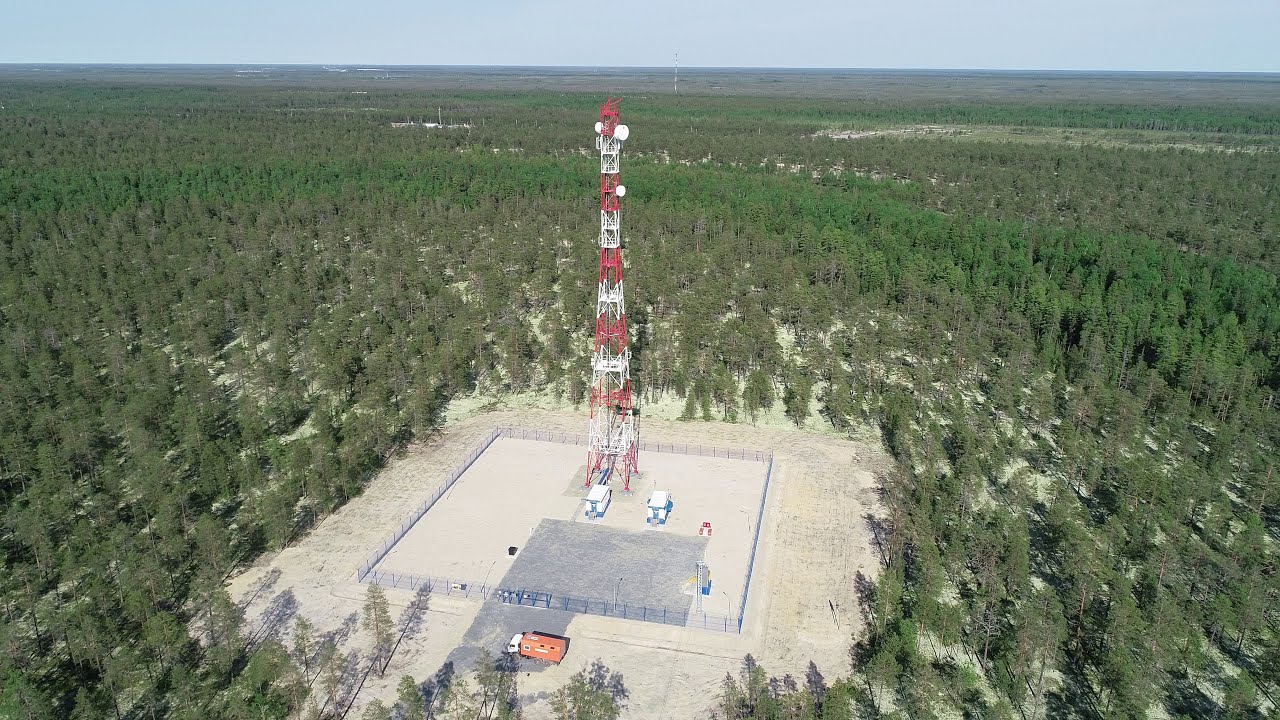This aerial shot captures a vast, flat expanse dominated by grassy and wooded areas stretching across the entire image. In the foreground, a large square plot stands out starkly against the greenery. This plot appears to be a mix of cement and dirt and is marked by a tall, red and white tower, possibly a satellite or electrical tower. Encircling the tower is a tall blue wire fence, which encloses various smaller machinery pieces and two white containers with blue trim. Just outside the fence, near the entrance, a white and orange truck is parked. The area around the fenced plot transitions into a forested landscape with spaced trees, their green and brown hues contrasting with the grayish ground below. The backdrop of the image features more densely packed trees extending into the distance, where faint outlines of another tower and possibly hills or more forested areas with a bluish hue can be seen. The overall scene is dominated by natural elements, making the industrial plot a striking focal point in this aerial view.